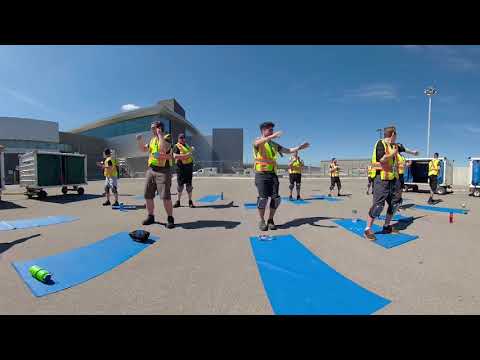In a spacious outdoor area, likely behind a warehouse or airport hanger, a group of approximately ten young men stands in a large circle on a flat, grey cement ground. Each man is wearing a neon yellow safety vest with red reflective straps, paired with dark-colored shorts and knee pads. They have their arms extended out in front of them, suggesting they are engaged in some form of coordinated activity or instruction. In front of each individual lies a long blue mat—resembling tarpaulin rather than yoga mats—scattered with various objects, including several water bottles in different colors. The scene is set against a bright blue sky, with a lamp post and cargo containers visible in the background.